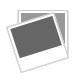The photograph captures an advertisement for roofing and siding by the Leehan Company, prominently featuring their association with Mulehide Products. The advertisement is a brochure-like placard resting on a background of brown shingles, which simulates the look of actual roofing material. At the top left corner of the sign, a rectangular section juts out with a red background and some unreadable white text. The main body of the sign has a white background with black text that includes an arrow pointing to the right and the words "Roofing and Siding" along with "The Leehan Company." Adjacent to this, there is a yellow circle outlined in red, displaying the Mulehide Products logo with a black mule mascot and additional text below it. The lower section of the sign transitions into a design resembling green vertical siding. To the left, there is extensive information about additional products such as bathroom vanities and cabinets. The entire setup resembles a packaged piece of roofing material, partially covered to reveal the branding and descriptions in multiple languages, possibly indicating international availability. The advertisement combines visual elements of both roofing and siding materials to enhance its appeal.